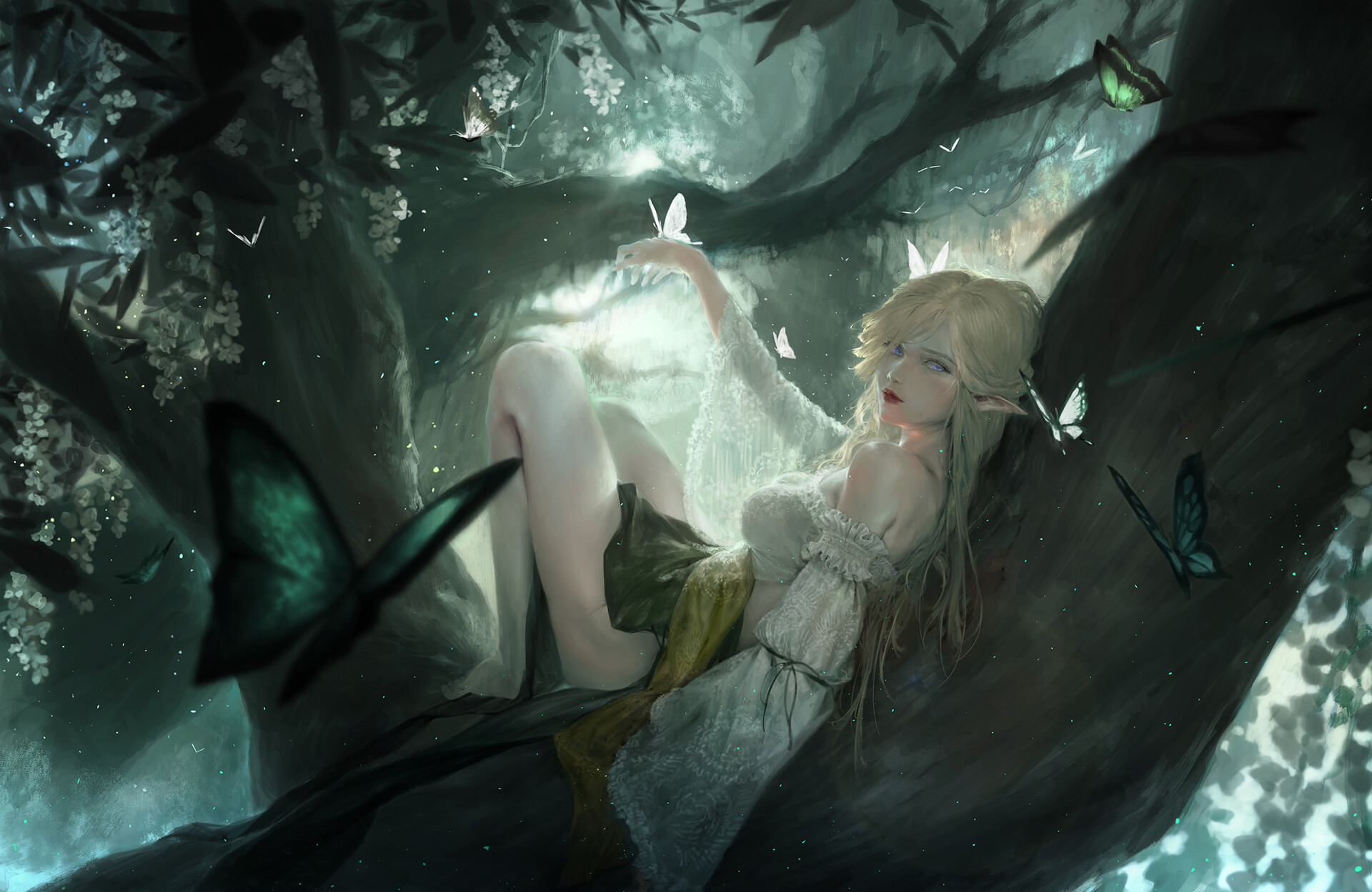The image depicts a detailed artistic rendition of a whimsical fae figure, lounging seductively on a dark brown willow tree branch, bathed in ethereal light filtering through the forest canopy. The fae, with striking blonde hair and vivid red lips, exudes an enchanting aura, accentuated by her white blouse, green skirt, and yellow wrap. The scene is awash with a palette of teals, whites, greens, and darker hues, creating a magical ambiance. She interacts with her surroundings as a white butterfly gently rests on her hand, while other butterflies—green, blue, and another white—flutter around her, adding to the fairy-tale charm. This captivating fae, occupying the central portion of the image, gazes alluringly towards the viewer, with an aura of mystery glowing from behind her.